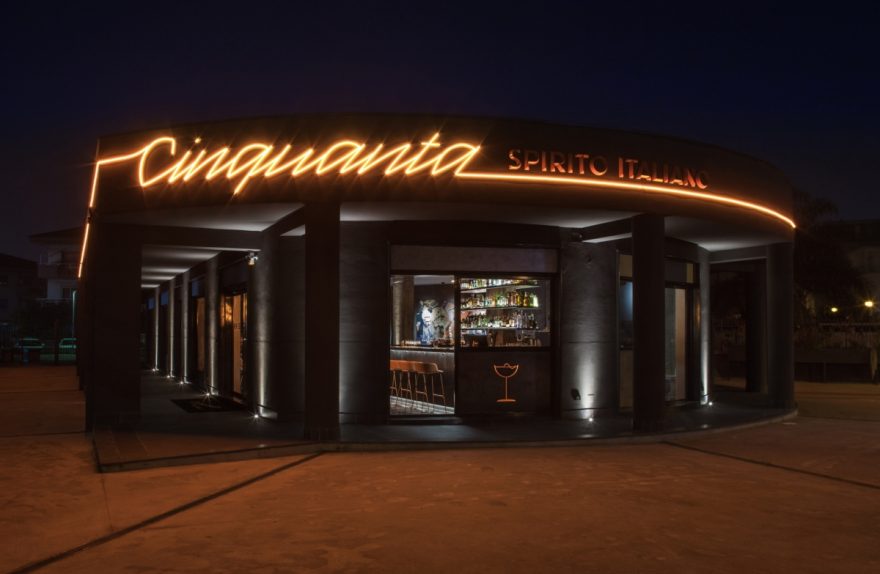This photograph captures the front entrance of a modern, black-painted bar and restaurant named Cinquanta, taken at night. The image is a horizontal rectangle, showcasing the sleek, open-air design of the venue with no visible doors. The building features a shiny black facade accented by white LED lights that highlight various parts of the exterior. Above the front door, a neon orange cursive sign spells out "Cinquanta," with a long LED light extending around the entire structure, emphasizing its sleek, circular shape. Directly beneath this, on a gold placard, is the secondary name "Spirito Italiano." The ground appears to be reddish-brown concrete, illuminated by the building's lights. The front door is open, and through it, brown chairs and bar stools are visible. The sidewalk, with a reddish-brown hue from the reflected lights, leads to a mixed drinks display to the left. An image of a martini glass decorates the front, further indicating the establishment's focus as a trendy bar. The building's windows extend along a long hallway on both sides, enhancing the welcoming and open atmosphere of this chic nighttime locale.